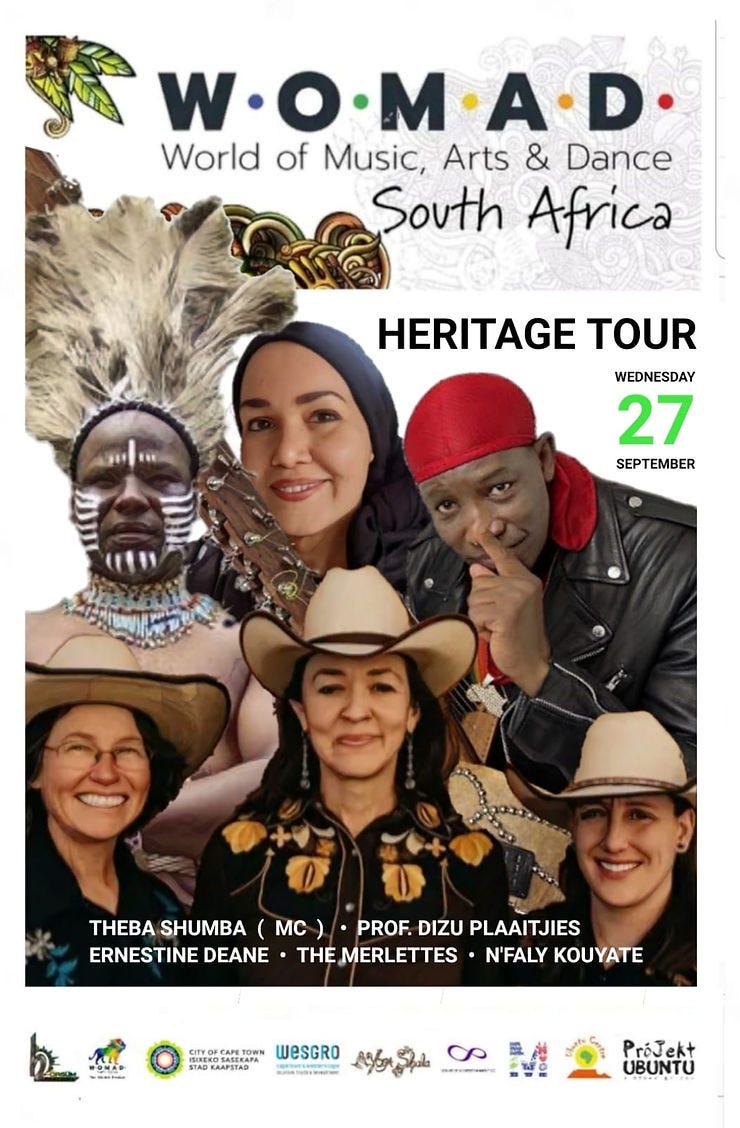The poster is a colorful advertisement for the WOMAD (World of Music, Arts, and Dance) South Africa Heritage Tour, taking place on Wednesday, 27th September. The event title, "WOMAD," is prominently displayed at the top with each letter accompanied by a dot of a different color (W in blue, O in green, M in yellow, A in orange, and D in red). Below the event title, the phrase "World of Music, Arts, and Dance, South Africa" is written, followed by "Heritage Tour."

The vibrant and lively poster features images of various performers. It includes a traditional African tribal member adorned with white feathers and face paint, a black man with a red headwrap and a significant beaded necklace, a woman with a black scarf around her head showcasing her hair, and three women dressed as cowgirls in matching cowboy hats and black shirts.

Beneath the performers' images are the names of the participants: Diba Shumba MC, Professor Dizu Plaatjies, Ernstine Dian, The Merlettes, and The Folly Kool-Aid. Additionally, the bottom section of the poster lists the event sponsors with their corresponding logos. The overall design exudes a vibrant and festive atmosphere, encapsulating the diverse cultural celebration of the WOMAD Heritage Tour.